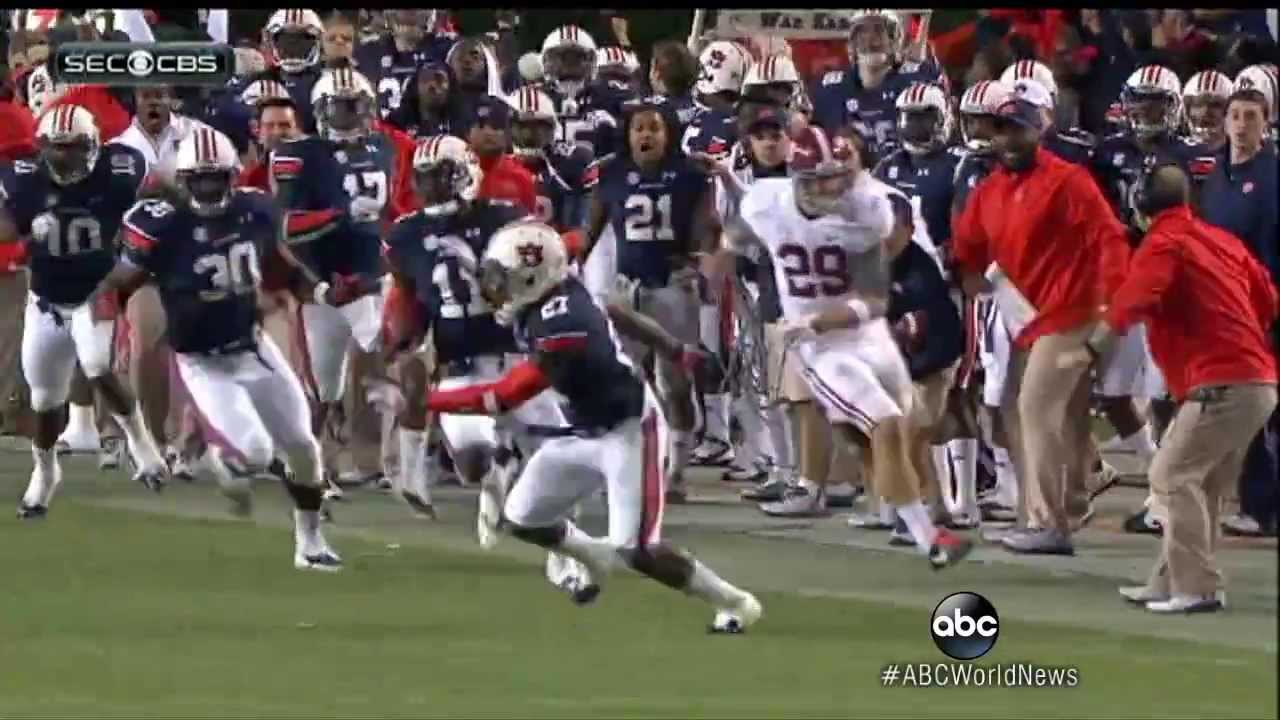The image captures the intense moment of a live American football game, viewed from an on-field perspective, possibly from the end zone angled towards one of the sidelines. One prominent player is darting across the field to the left, while others from his team, clad in blue and white jerseys with red accents, are gathered on the sidelines with surprised or excited expressions. Opposing players, who wear mostly white jerseys with red numbers and helmets, are also in motion, particularly one running along the edge of the sidelines. Coaches in red shirts with headsets, one appearing to shout instructions, are actively engaged close to the sideline. The scene is vibrant with motion and emotion, underscored by broadcast graphics—'ABC World News' in the bottom right corner and 'SEC' along with 'CBS' in the top left—highlighting its coverage as a significant event. The players' jerseys and team colors, blue with red and white for one team and white with red for the other, alongside the shared detail of white pants and distinctive helmet designs, further enrich the vivid storytelling of this football game captured at a climactic moment.